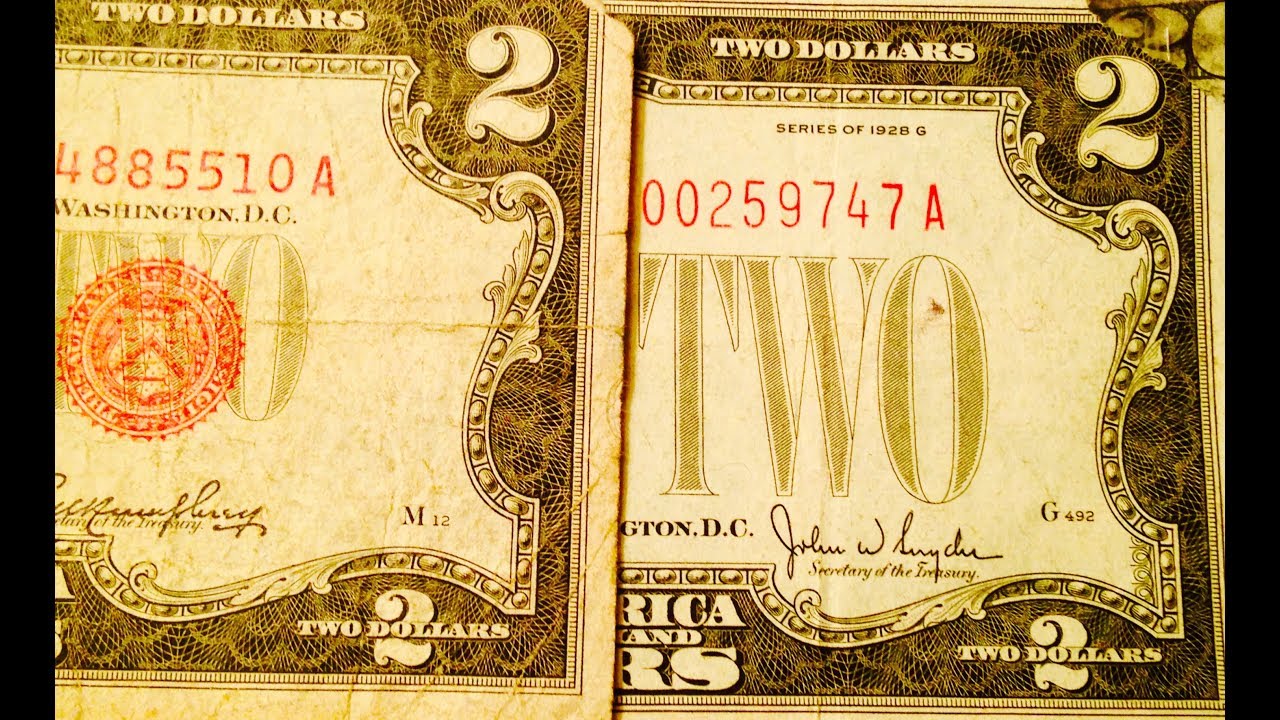The image depicts two $2 bills horizontally aligned against a solid black background, with the left bill appearing older and more faded, displaying a yellowed hue. Both bills are partially visible, with one overlapping the other. The left bill shows the right side, featuring the number "2" in the top and bottom right corners, and the red serial number "4885510A" along with "Washington, D.C." beneath it. This bill has a distinctive red stamp across it and also includes the designation "M12" in black lettering.

The right bill appears clearer and greener, indicating it is better preserved. It is flipped upside down, showing the serial number "00259747A" in red text, and the series inscription "Series of 1928 G" at the top. The bill sports the large word "TWO" in the center, similar to the older bill, and has a red stamp across it. The right bill also bears the designation "G492" in black lettering. Both bills have signatures and maintain a consistent design, although the preservation state differs significantly between them.